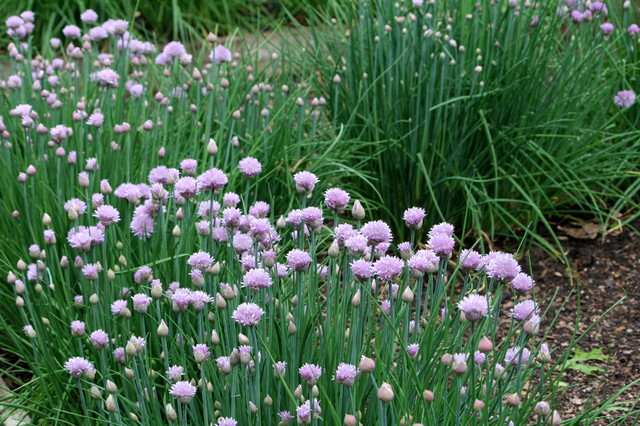In this spring evening scene, we see a cluster of tall, stringy, grassy allium plants—possibly chives or wild garlic—standing in a yard with moist, enriched, dark soil that is speckled with lighter shades of brown and cream. These plants are arranged in a row that curves toward the foreground of the image. The vibrant purple flowers, some in full bloom with tightly clustered petals, add a splash of color. Other blooms remain coiled in bulbs, hinting at ongoing growth. Bright lavender and light lavender hues dominate the blooming flowers. In the background, undeveloped buds contrast with the vibrant front, suggesting the vast, plentiful spread of these plants. A sidewalk or pathway is seen behind the plants, possibly indicating a park-like setting with further greenery beyond.